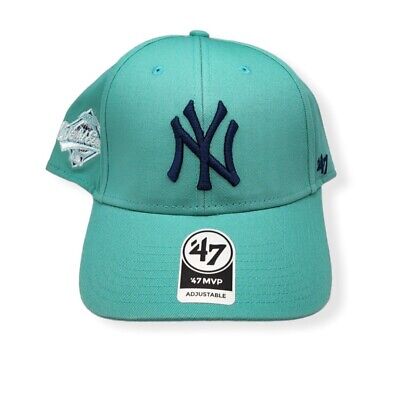The image depicts a New York Yankees baseball cap, prominently featuring a dark blue "NY" logo embroidered on the front, with the "Y" interwoven on top of the "N." The cap is an aqua blue color, adding a unique touch compared to the traditional team colors. A sticker labeled "47" is affixed to the brim, with black text on a white background reading "47 MVP" and "adjustable," indicating the cap's adjustable size feature. The cap exhibits professional detailing, including three visible lines—one down the middle and one on each side. Additionally, the left side of the cap displays a partly visible emblem related to the World Series, while the right side has some unreadable black text. The photo is set against a pristine white background, enhancing the sharp, professional lighting and faint shadows that create a 3D effect, emphasizing the cap's contours.